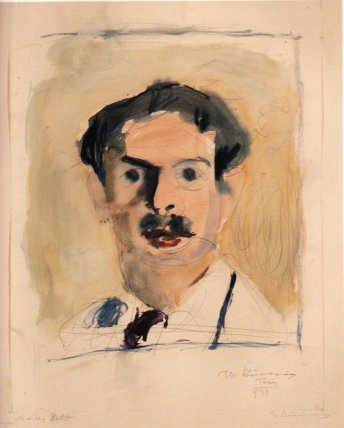This image is an impressionistic, possibly watercolor, painting of a man on tan-colored paper. The background is a blend of beige, orangish, and greenish tones, with hints of a faint, broken gray frame along three edges. The man has dark black hair, deeply prominent black eyes, a thick black mustache, and burgundy red lips. His nose is aquiline, casting shadows that extend over his right eye. He wears a white shirt with a black tie and a thin black line that could suggest a suspender on the right side, and a blue spot on his left shoulder. The image conveys a loose, impressionistic style with minimal lines and shapes, and captures the face of the man with a sort of shocked or alarmed expression. Additionally, the artwork is signed in two places, although the signatures are in pencil and not legible.